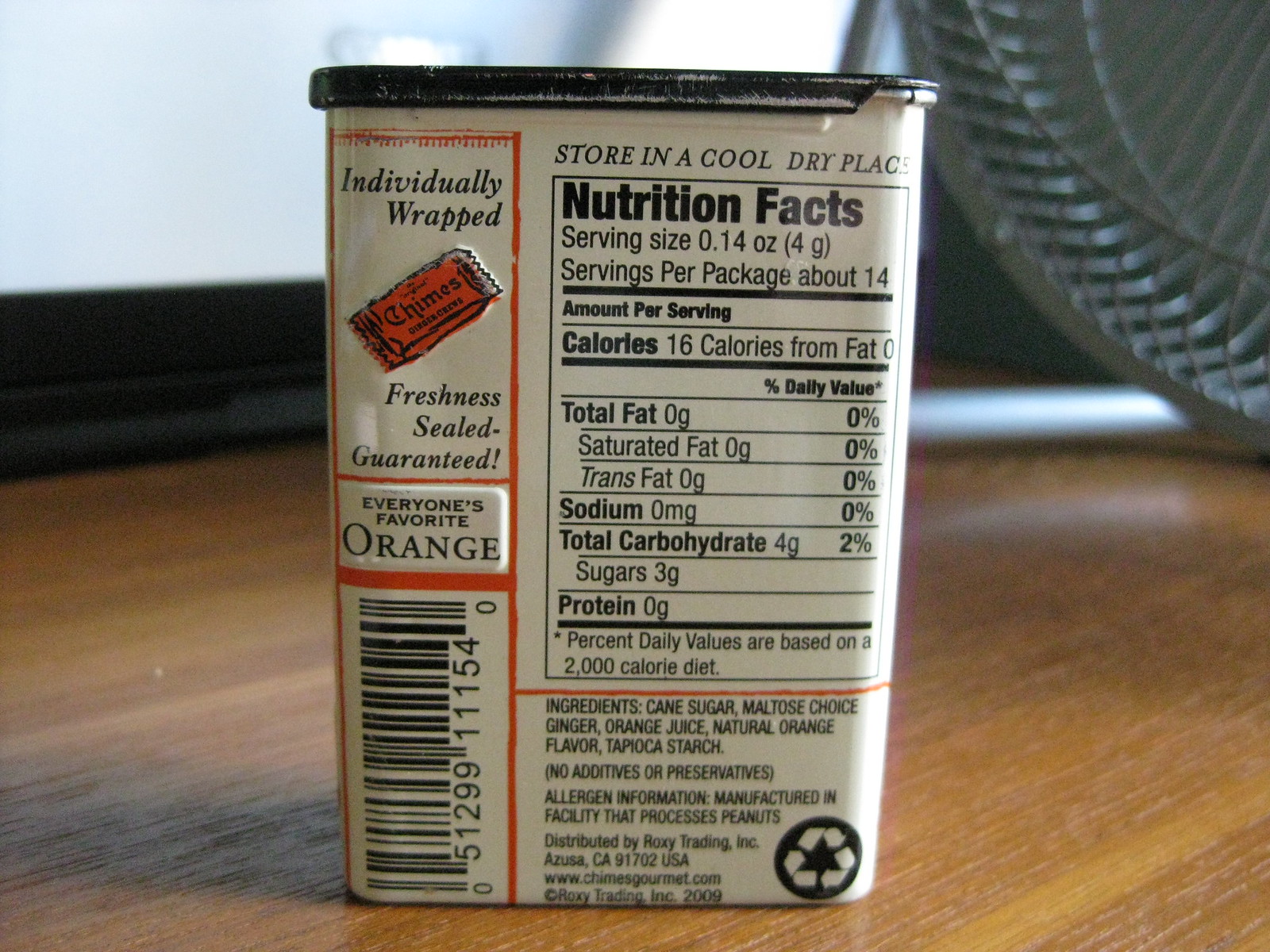The photograph depicts the back of an oval-shaped metal candy tin with a black lid, positioned on a brown floor against a wall that has a white upper portion and a black lower portion. The tin, featuring a red border and some white scratches, showcases various texts and graphics. The top left corner reads "Individually wrapped, freshness sealed, guaranteed." Below this, "Everyone's favorite, orange" is printed, along with an image of an orange-wrapped candy. A UPC code is located beneath this text, set against an orange highlight. The right side of the tin displays the nutrition facts, listing ingredients such as cane sugar, maltose, ginger, orange juice, natural orange flavor, and tapioca starch. There is an instruction to "Store in a cool, dry place" in the top right corner. The background includes a circular, grey object resembling a fan in the upper right corner, suggesting the setting might be on the floor near a cooling fan.